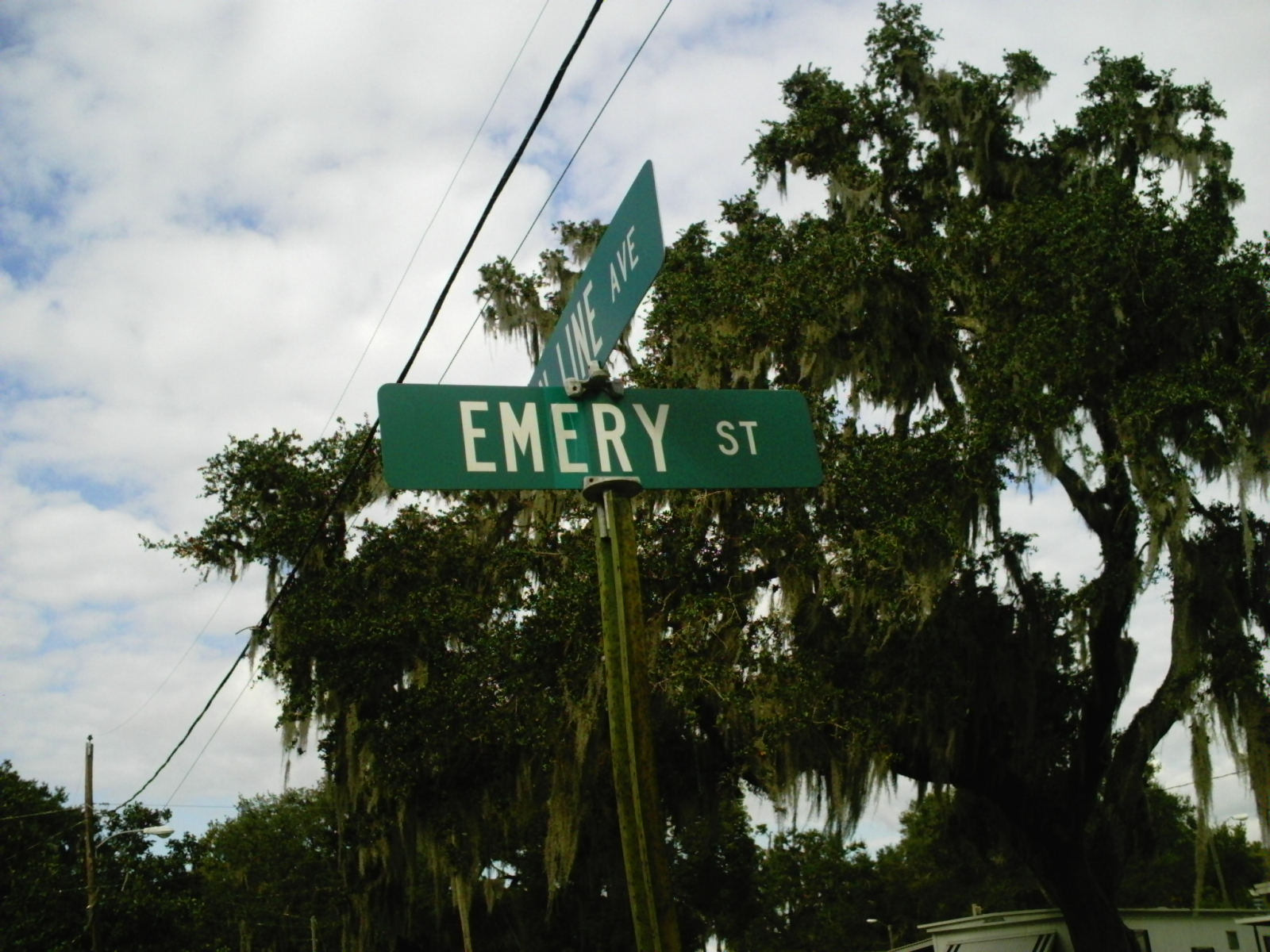The photograph showcases a single street sign in the center, prominently featuring green metal signs mounted on a slightly rusted pole. The visible sign reads "Emory Street" horizontally, spelled E-M-E-R-Y, while the top sign, positioned slightly at an angle, partly displays "Rhine Avenue." In the background, large, wispy willow trees stretch their branches outward, and a power line extends from the top left corner across the scene. Above, the sky is predominantly filled with white fluffy clouds, with hints of blue peeking through.